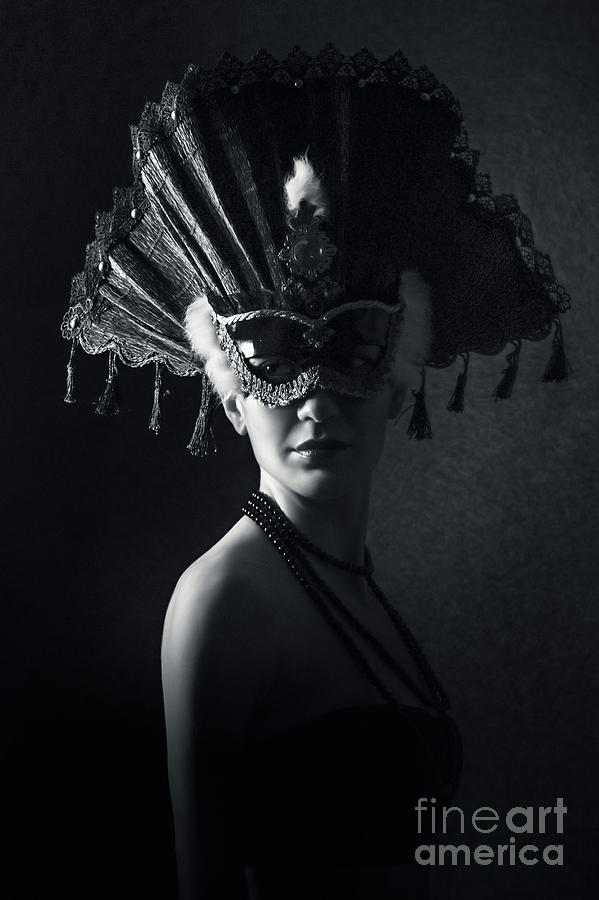This black and white photograph captures a striking image of a young woman, likely in her early twenties, with short blonde hair. She is elegantly dressed in a strapless dress, adorned with a three-tiered pearl necklace that drapes gracefully around her neck. The high-contrast photograph shows her in the center of the frame with her right shoulder in the foreground and her head turned towards the right, casting an enigmatic gaze directly into the camera. 

Her visage is partly concealed by an elaborate masquerade mask, reminiscent of a turn-of-the-century ball accessory. The mask, ornate and eye-catching, only covers her eyes and features a large, fan-like headpiece adorned with jewels and tassels that hang from its edges, enhancing its grandeur. The light source from the left illuminates her mask and upper torso, creating a dramatic interplay of light and shadow, while the background remains dark. 

This artwork, evocative of an old-fashioned yet timeless elegance, is accompanied by the text "Fine Art America" in the lower right corner, suggesting it is a purchasable print from this company. The overall composition, with its meticulous detail and sophisticated aura, makes the photograph a visually captivating piece.